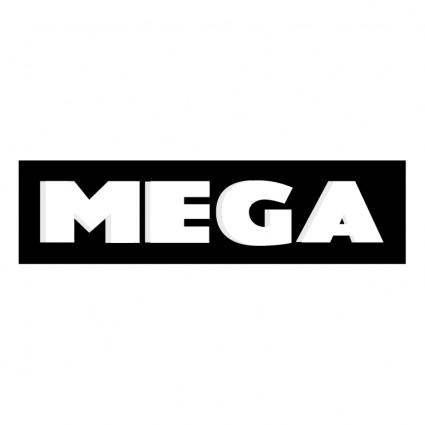The image features a centrally positioned black rectangle on a white background. Within the rectangle, in large, bold, and boxy white letters, it spells out "MEGA." The letters are all caps and horizontally aligned, with the M, E, and A being particularly wide. The A has a distinctive, short, triangular cutout. The lettering is centered perfectly within the black rectangle, and there are no additional images, text, or shadowing effects. The overall design is straightforward, comprised solely of the contrasting colors black and white.